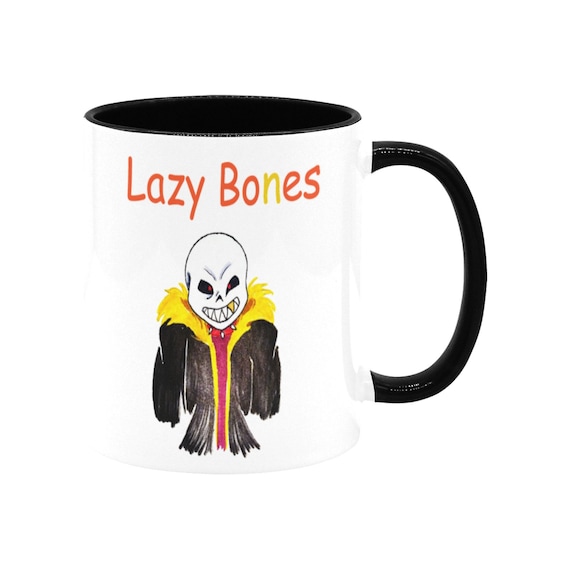This image portrays a coffee mug designed with distinct and vivid details. The mug itself features a striking contrast with a white exterior, black interior, and a matching black handle. Prominently displayed at the top in thin red font are the words "Lazy Bones," with the letter 'N' in "Bones" uniquely colored in a yellow-orange hue. Below this text is a detailed illustration of a grinning skull. The skull's eyes are deeply hollow and dark, exuding an eerie yet playful demeanor, with one tooth gleaming gold among its otherwise white, dagger-shaped teeth. The skull is dressed in an eclectic outfit consisting of a black jacket adorned with a yellow fur-lined collar and a red shirt underneath. A tri-pointed bone necklace adds to the skeleton's quirky style. The intricate design and bold colors make this coffee mug visually captivating.